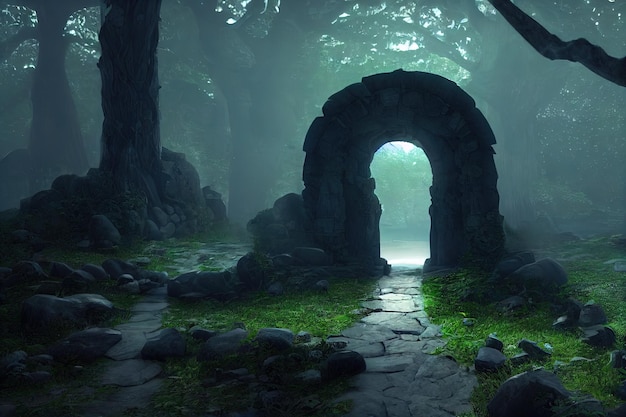In a hazy forest filled with towering trees, there's a prominent stone archway standing alone, giving the scene a mystical atmosphere. The arch, crafted from smooth, flat gray stones, forms a passageway leading to an area shrouded in mist. Surrounding the arch on both sides, the lush green grass appears slightly overgrown, adding to the untamed, natural beauty of the scene. 

In front of the arch, there are numerous piles of mostly round, gray rocks scattered randomly, enhancing the rugged feel of the landscape. As you look through the arch, a gentle light penetrates the fog on the other side, revealing hints of vibrant green. The trees flanking the pathway are massive, with thick trunks and dense, leafy branches that obscure much of the view.

Additionally, there is a narrow path to the left made of a single line of flat stones, providing a secondary route within this enchanting setting. The overall atmosphere, with its foggy haze and ethereal qualities, evokes a sense of stepping into a fantasy world.